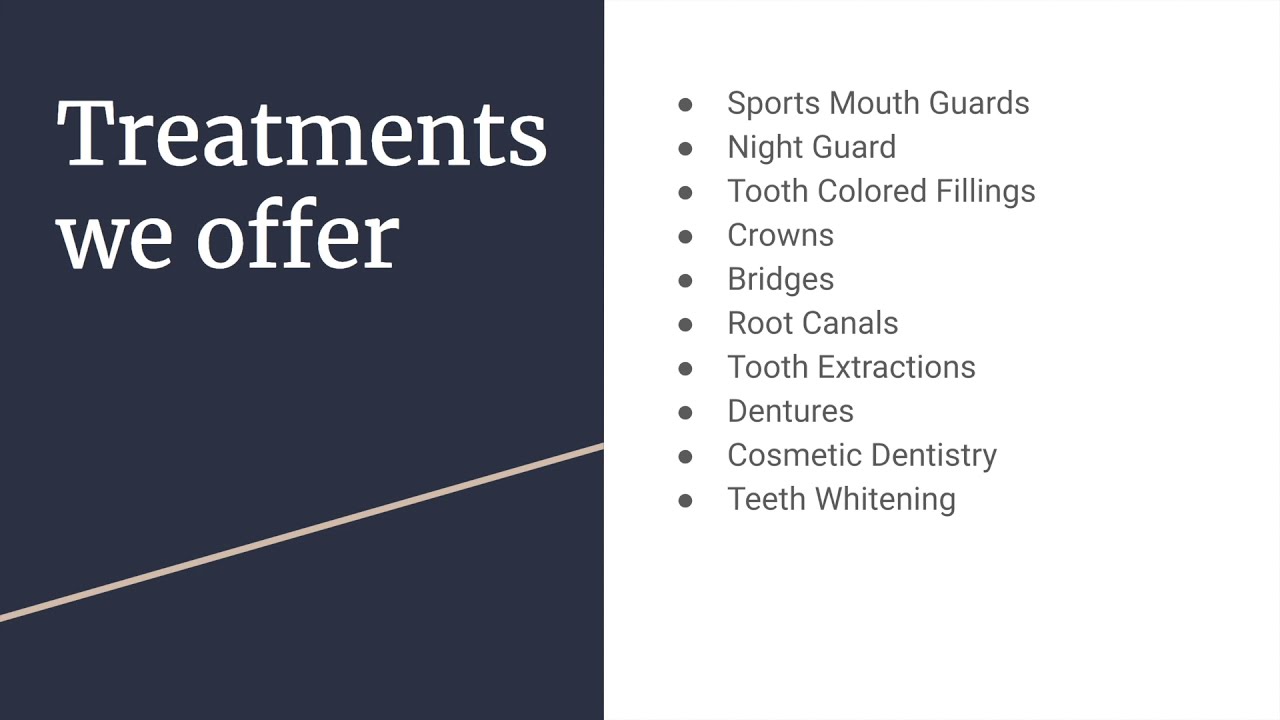The image is a detailed advertisement for a dental office, resembling a presentation slide or poster. The left side features a dark navy blue or dark gray rectangle with a white or tan diagonal stripe near the bottom. At the top of this rectangle is a white serif headline that reads "Treatments We Offer." To the right, on a white background, is a bulleted list of treatments written in dark gray or black text. The bullet points, which are small circles, enumerate the treatments offered: sports mouth guards, night guards, tooth-colored fillings, crowns, bridges, root canals, tooth extractions, dentures, cosmetic dentistry, and teeth whitening. This precise layout presents the services in a structured, visually appealing format. The rest of the image is uncluttered, maintaining a clean and professional look.